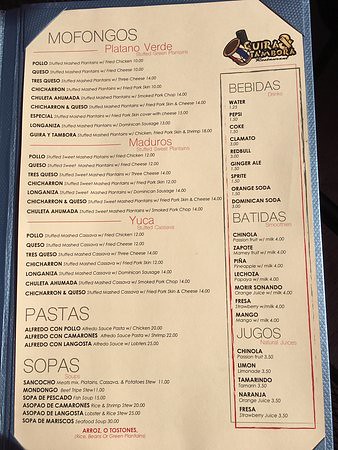This is an image of a restaurant menu, primarily written in Spanish, although some parts are partially unreadable. The menu is divided into several sections with different food offerings.

The top section of the menu is somewhat unclear, but it appears to have the name of the restaurant, which might be "Guira Tambo" or a similar name.

On the left-hand side, the first section lists various dishes with the heading "Plátano Verde." Some of the items in this section include:
- Pollo (Chicken)
- Guiso (Stew)
- Tres Quesos (Three Cheeses)
- Especial Longaniza (Special Longaniza Sausage)

The next section is shaded in a pinkish color and it lists dishes under "Maduros" (Sweet Plantains). The items here include:
- Pollo (Chicken)
- Queso (Cheese)
- Tres Quesos (Three Cheeses)
- Chicharrón (Fried Pork Skin)
- Longaniza (Sausage)

Following this, another pinkish section is dedicated to "Yuca" (Cassava) dishes with items like:
- Pollo (Chicken)
- Various other items building on the base ingredient yuca.

Below the yuca section, there is a pasta section featuring three pasta dishes, and further down, a soup section ("Sopa") offering six different types of soups.

On the right side of the menu, there is a beverages section labeled "Bebidas," which likely includes drinks. The visible options in this section are water, Pepsi, Coke (Coca-Cola), and jugos (juices).

This detailed breakdown attempts to capture as much information as possible from the partially legible text in the photograph.